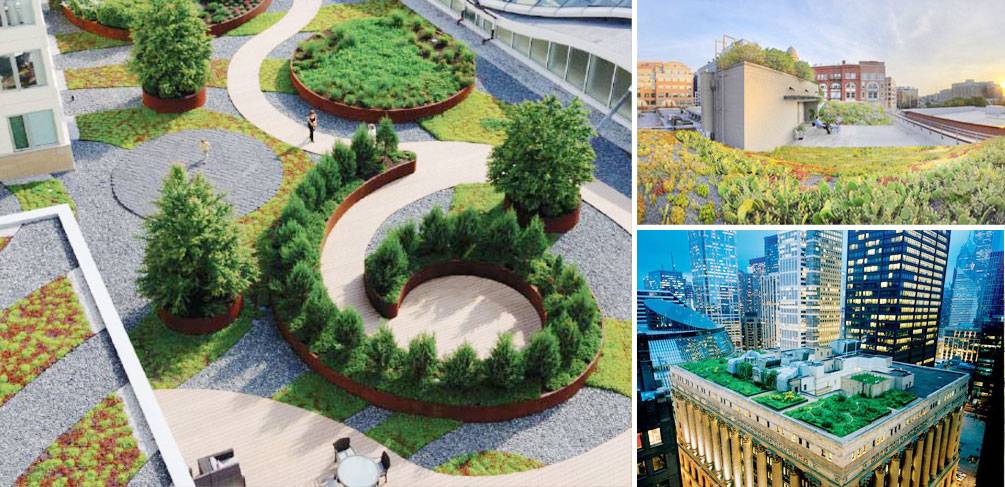This image collage is divided into three sections: the larger left section and two smaller sections on the right, arranged vertically. The left section, which occupies two-thirds of the collage, features an aerial view of a meticulously manicured rooftop garden with swirling pathways lined with evergreen bushes shaped to form the number six. Interspersed throughout the design are other plants set in various pavement sections, all bathed in bright sunlight. The top right section showcases another perspective of this garden with a view of surrounding city buildings and additional greenery in the foreground under a sunny sky. Notable structures include a small tan building in the center and red brick and tan buildings in the background. The bottom right section switches to a nighttime scene, capturing an illuminated cityscape with skyscrapers. The viewpoint is from another rooftop garden, which appears to house plants and possibly small structures, offering a serene, urban retreat above the bustling city.